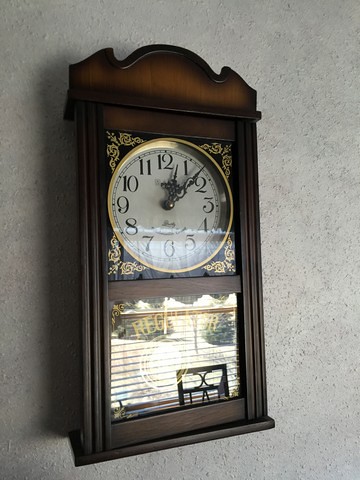This photograph captures a rectangular, dark-stained wooden wall clock set against a textured light gray stucco wall. The sunlight streaming from the right side of the image casts a faint shadow to the left of the clock. The clock, framed by a slightly ornate wooden box with gold filigree and wave-like detailing at the top, is richly dark brown with a gold trim encircling a white clock face. Black Arabic numerals, a pair of elegant, black metal hands with swerve designs at the tips, mark the hours and minutes; there is no second hand present. The face of the clock is framed by a gold rim and set within four gold-detailed corners forming triangular shapes between the circular inset and the square outline of the clock. Below this section is a glass pane reflecting a living room chair and window blinds from the background, slightly obscuring any potential lettering in gold on the glass. The pendulum is faintly visible through the reflective glass at the bottom, hinting at its rhythmic motion. The clock displays the time as 12:08.